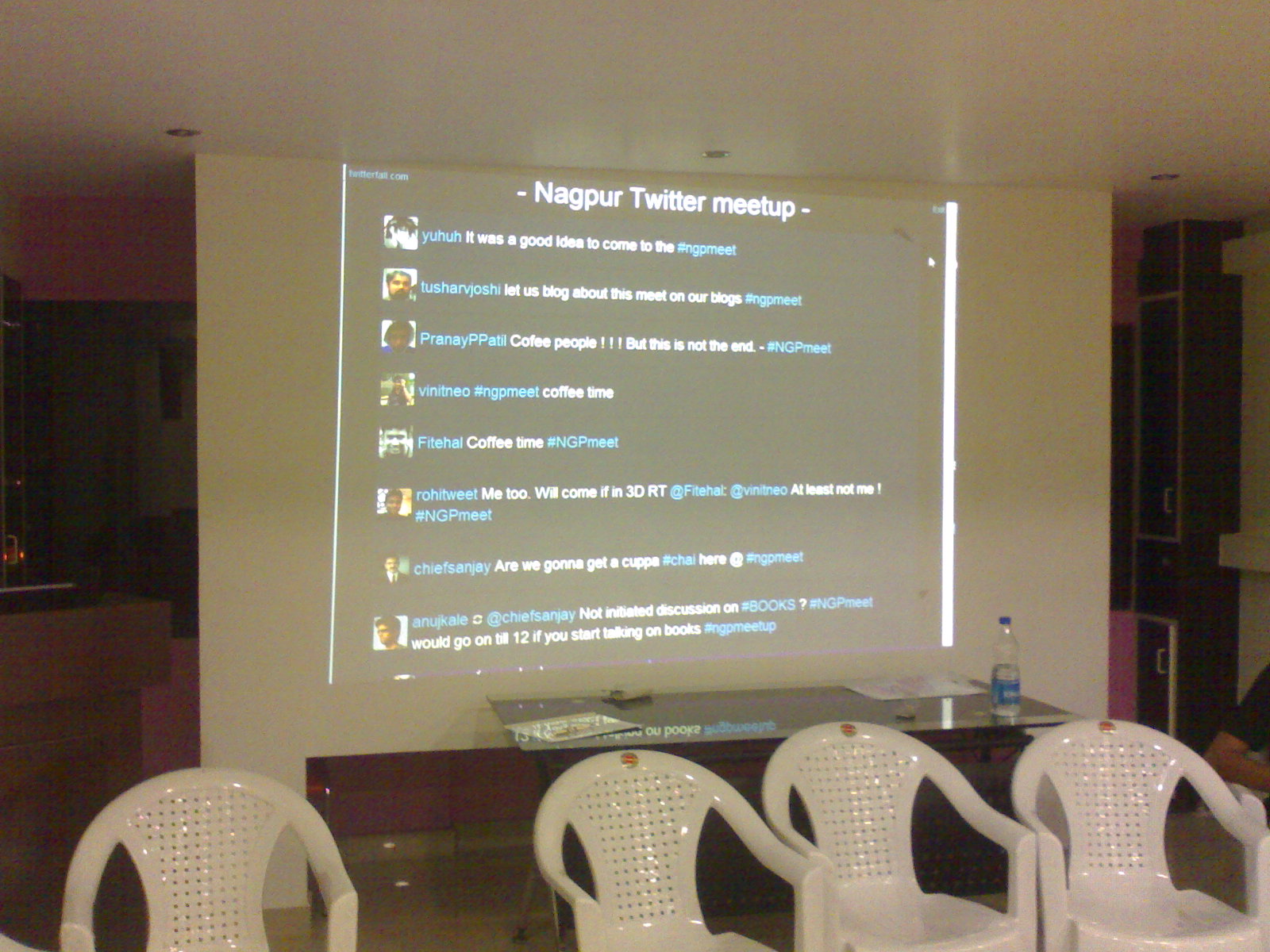In a room with a brown floor and white or black cabinets on the right, there is a large green screen displaying a projected image. In front of the screen, there is a green table with a bottle of water on the right side and four white plastic chairs facing the screen. The screen prominently features the text "Nagpur Twitter Meetup" at the top, followed by a series of tweets and profile pictures from various participants. The tweets include messages such as "It was a good idea to come to the #NGPmeet," "Let us blog about this meet on our blogs #NGPmeet," "Coffee people! But this is not the end #NGPmeet," "Coffee time #NGPmeet," "Me too, will come if in 3DRT at least not me! #NGPmeet," "Are we going to get a cup of #chai here #NGPmeet," and "Not initiated discussion on #books? #NGPmeet would go on till 12 if you start talking on books." The room is set up to host what appears to be a discussion or presentation centered around the tweets displayed on the screen.